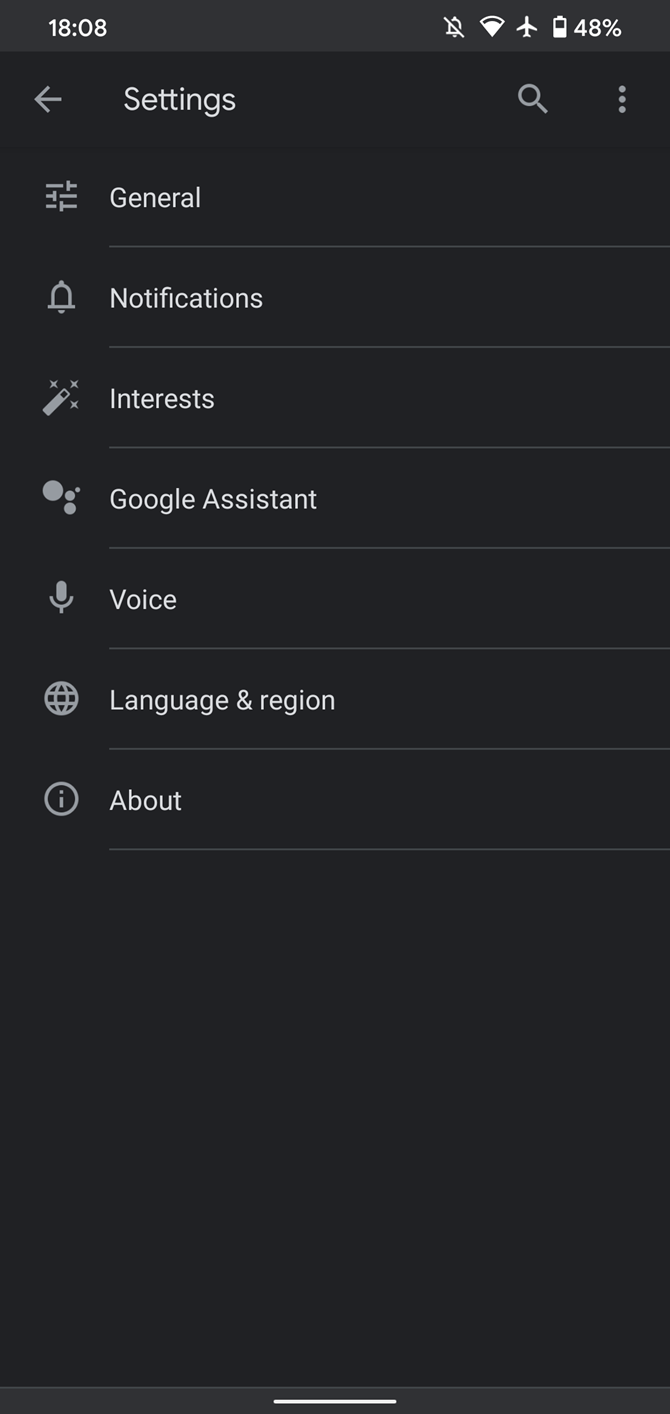The image depicts the settings section of an Android-style phone as viewed on a mobile device. At the very top, a gray banner displays white text and icons. On the left side of the banner, the time reads "18:08." A series of icons follow this, including a notification icon with a cross through it, indicating notifications are disabled, a nearly full Wi-Fi signal icon, an airplane mode icon, and a half-charged battery icon showing 48% remaining. 

Below this banner, on a black background, there is a gray arrow pointing left, likely serving as a back button. The title of the page, "Settings," is prominently displayed. Adjacent to the title, there's a search bar for finding specific settings and a More Options button represented by three vertical dots. 

The settings list below is categorized into various sections:
1. **General** - Icon: Filter button
2. **Notifications** - Icon: Bell
3. **Interests** - Icon: Magic wand
4. **Google Assistant** - Icon: Bubbles
5. **Voice** - Icon: Microphone
6. **Language and Region** - Icon: Globe
7. **About** - Icon: Eye within a circle

Each section is clearly labeled with its respective icon to the left, making navigation straightforward.